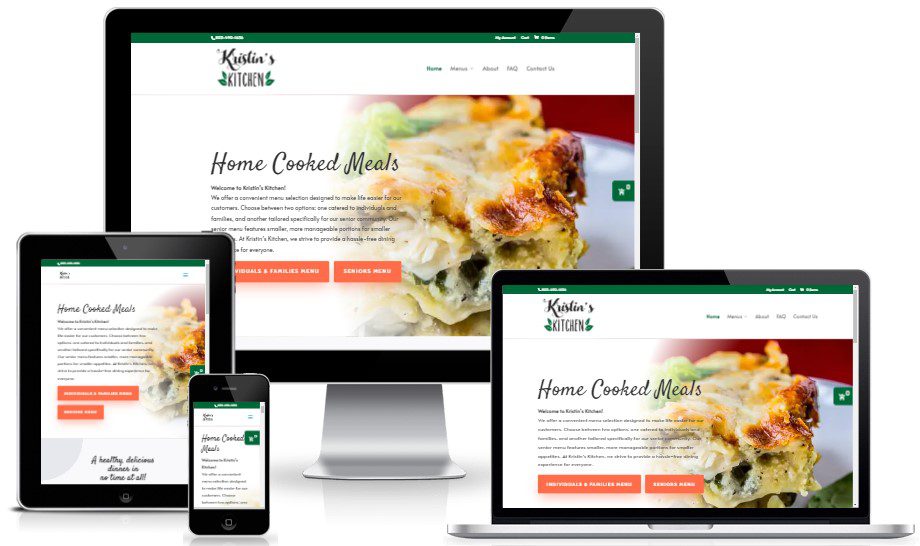This image showcases a responsive website design for "Kristen's Kitchen" displayed across various Apple devices. In the background, an Apple monitor highlights the website with a clear green header and a menu on the right side. In front of the monitor sits a MacBook Pro, presenting an identical view of the site.

On the left, an iPad is placed vertically, displaying the website with vertically stacked orange buttons beneath a partial hero image of a delicious, close-up shot of lasagna, emphasizing its thick, cheesy layers. Slightly in front of the iPad and to its right is an iPhone. The iPhone version also shows the green header and scripted "home-cooked meals" text but omits the hero image and buttons due to its smaller screen size.

The website features a hero image of food fading into a yellow background which contains text and two orange buttons. Across all devices, the scripted "home-cooked meals" text and logo remain consistent, although the layout adapts to fit each screen size accordingly. The display includes realistic drop shadows and a shiny surface effect, enhancing the presentation's visual appeal and coherence.